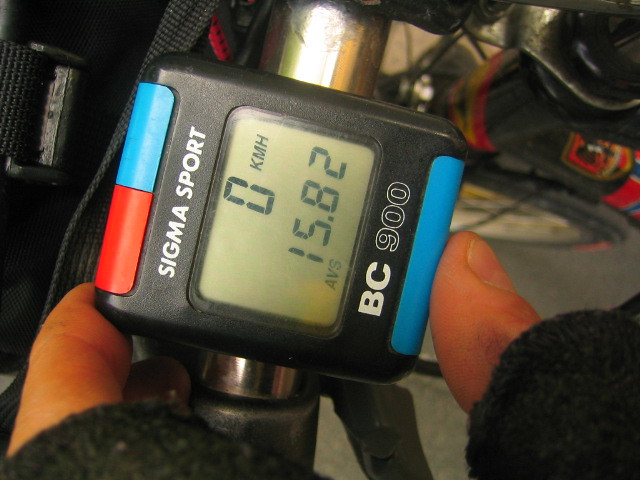In this photo, we can see a close-up view of a cycle computer attached to the handlebars of a bicycle. The device features a small rectangular display that shows the current speed as "0 KMH". Below this, the display reads "AVS 15.82", indicating the average speed. The top of the device has two buttons: a red button on the left and a blue button on the right. In white text above these buttons, the brand name "Sigma Sport" is clearly visible. At the bottom of the cycle computer, there is another blue button, and the model indication "BC 900" is marked in black font with a white outline on the black surface. In the picture, a hand is reaching out to hold and properly position the device, which is mounted on the metal railing of the bike’s handlebar. The background reveals a part of the bicycle frame in the upper right corner, which is black and adorned with red and yellow stickers.